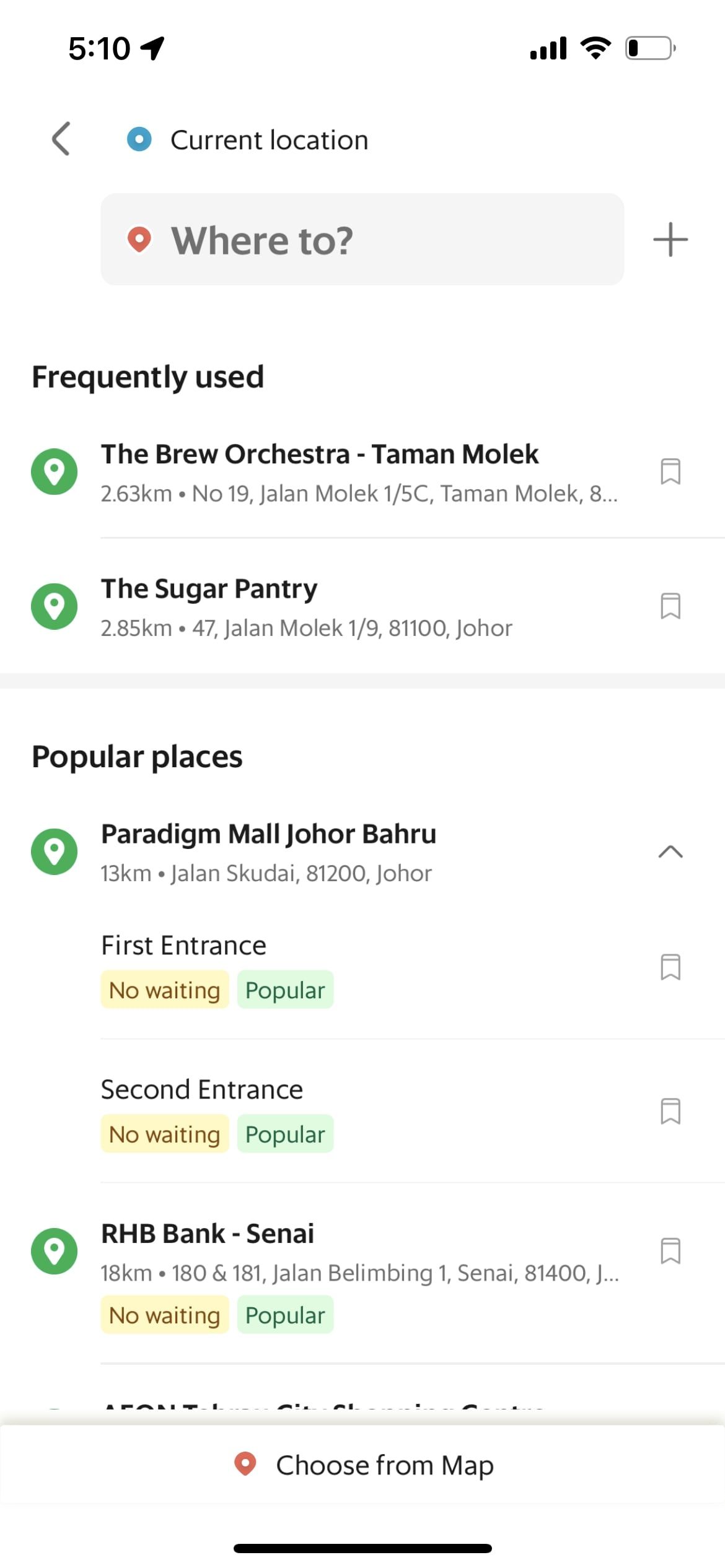The image is a vertical mobile screenshot taken on a phone at 5:10 PM. It reveals the phone has full service and active Wi-Fi, but the battery is at about 20%. At the top of the screen, it displays "Current location" and features a gray search bar with the prompt "Where to?", showing a red location icon and a plus sign on the right.

Below the search bar, the text "Frequently used" appears in black. The top search result is "The Brew Orchestra, Taman Molek," located 2.63 km away at 19, Jalan Molek 1/5C, Taman Molek. It has a green circle with a white location icon next to it. Following that is "The Sugar Pantry," 2.85 km away at 47, Jalan Molek 1/9, 81100 Johor.

Underneath the frequently used section is "Popular places," which includes "Paradigm Mall, Johor Bahru," 30 km away at Jalan Skudai, 81200 Johor. It specifies "First entrance" with options for "No waiting" in yellow and "Popular" in green. The same options appear for "Second entrance." Lastly, there's a mention of "RHB Bank, CNI."